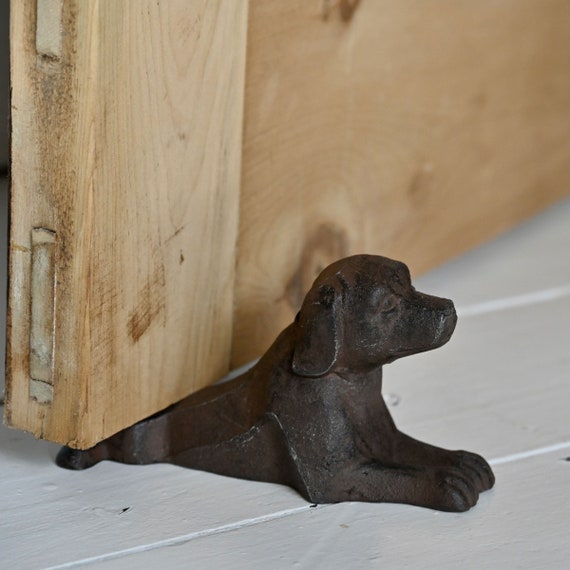The image showcases a charming, cast iron doorstop shaped like a small dog, most likely a labrador, with intricate detailing that emphasizes its endearing features. The dog is positioned as if casually lying down, with its front legs stretched forward and its head raised, mimicking a natural, relaxed pose. The back end of the dog is ingeniously crafted into a flattened wedge to effectively hold the door open. The door itself is made of rustic, unfinished light-colored wood, highlighting the natural wood grain, and exudes a vintage charm. The floor beneath is a lightly painted wooden surface, in a near-white hue with a hint of greyish blue, complementing the rustic aesthetic. This product photo clearly illustrates the practical use of the dog-shaped doorstop, while also focusing on the crafted details that make it an attractive gift for dog lovers.